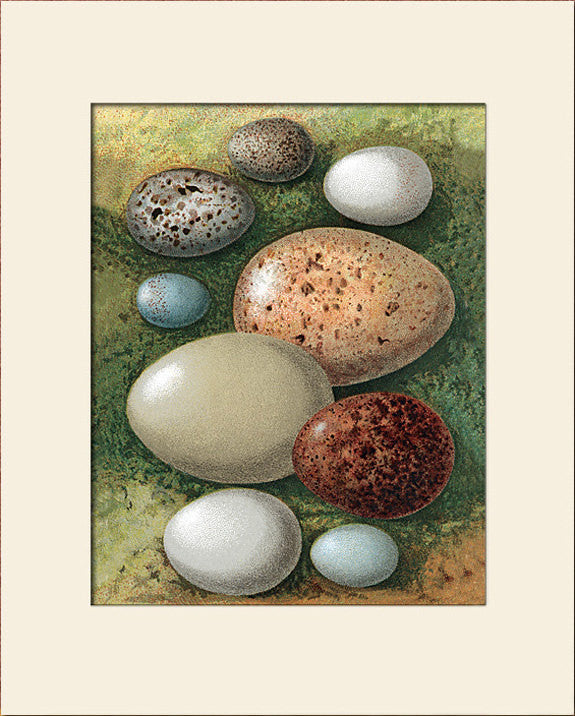This vertically aligned rectangular image, framed by a beige border, depicts an assortment of different colored and spotted eggs arranged on a grassy background. The grass transitions from darker shades in the center to lighter greens and browns at the top and bottom. In total, the image showcases approximately nine eggs of varying sizes and colors, each delicately shadowed to emphasize their three-dimensional quality.

At the center lie the three largest eggs: a solid tan egg, a slightly larger tan egg with brown spots, and a dark brown egg with even darker spots. Scattered among these are various smaller eggs, including two white eggs at the bottom and another in the upper right corner. The distinctive blue egg, likely a robin's egg, sits adjacent to the central large egg. In the upper left corner, two gray eggs adorned with brown spots complete the collection.

The diverse display includes eggs that resemble traditional chicken eggs and more exotic varieties, characterized by their unique speckled patterns and vibrant hues of blue, gray, maroon, and orange. The overall composition artistically captures the beauty and diversity of eggs set against the richly textured backdrop of interwoven greens and browns, making this piece a detailed and captivating study of nature's variety.